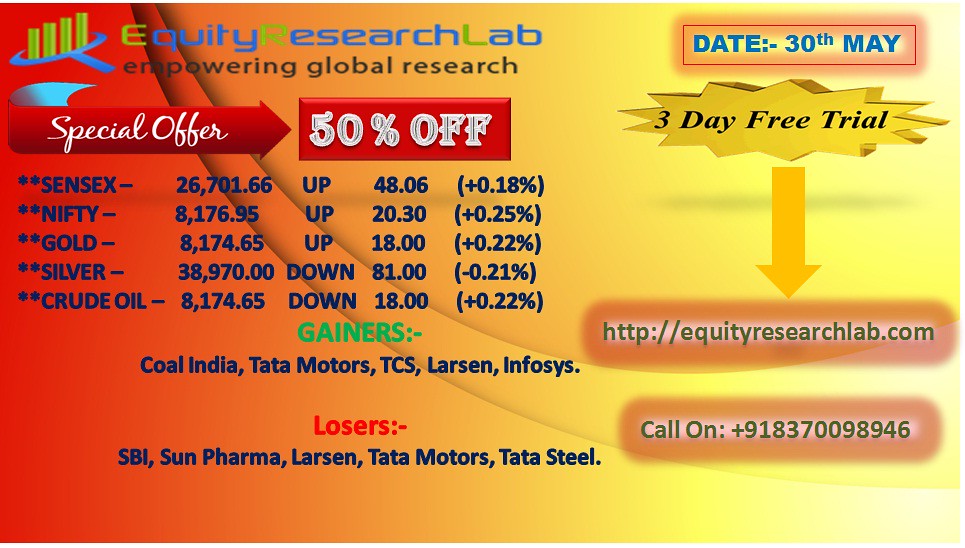The advertisement for Equity Research Lab presents a vibrant background that transitions from dark blood orange on the left to pale yellow on the right. Dominating the top left corner, the company logo features a stylized magnifying glass with four green columns emerging from it, adjacent to the title, "Equity Research Lab: Empowering Global Research." Below this, a prominent red arrow with the text "Special Offer" points towards a ribbon stating "50% off." 

In the upper right-hand corner, the date "30 May" is displayed in blue letters within a block. Beneath this, a mustard-colored starburst touts a "Three-Day Free Trial," followed by a downward-pointing arrow leading to a URL and a phone number for further contact. 

The ad provides detailed financial information, including a list of five commodities—Sensex, Nifty, Gold, Silver, and Crude Oil—each displaying current prices and their respective gains or losses. Additionally, it enumerates five top gainer stocks in green, such as Coal India, Tata Motors, and Infosys, and five loser stocks in red, which include SBI, Sun Pharma, and Tata Steel.

Overall, this meticulously crafted advertisement emphasizes its special offer and presents comprehensive market data to attract and inform potential clients.